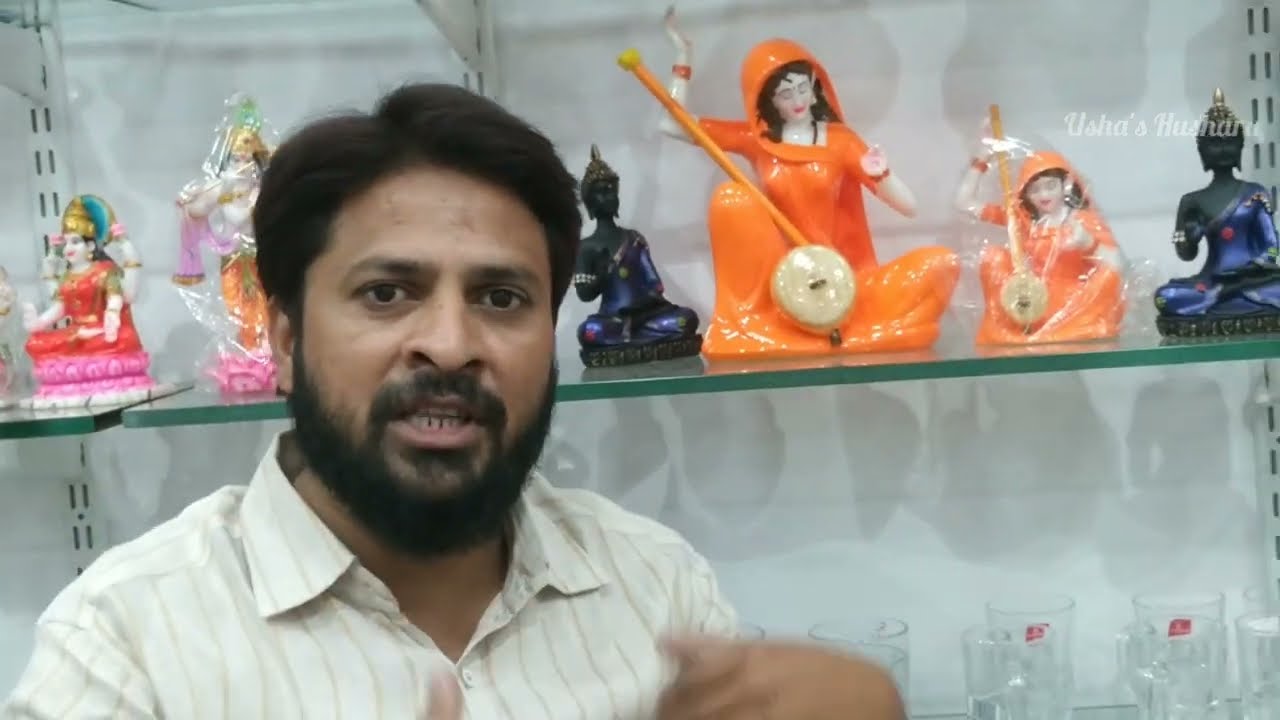In the foreground of the photograph is a middle-aged man, likely in his late 40s to early 50s, with brown skin and dark black hair that's neatly parted. He has a black mustache and beard and is wearing a white button-down shirt with thin blue stripes. The man is positioned on the left side of the image, shown from just below the shoulders to the top of his head, and he is in the midst of speaking, gesturing with his left hand raised slightly in front of his chest. 

Behind him is a stark white wall with a glass display shelf holding several ornate sculptures and figurines. To the left, a prominently featured figure appears to be an Indian goddess adorned in a red sari with a golden crown, standing on a pink base and accompanied by elements of blue. Moving towards the right, another figurine wears an orange sari, playing a stringed instrument, while further right, a black Buddha-type sculpture is visible. Additionally, there is a clear plastic-encased sculpture and another woman in a pink and red festive dress with an elaborate headdress. Lower down on the shelf, several glasses with red labels are also visible. All these elements suggest the setting of an artisanal shop filled with culturally significant artifacts.